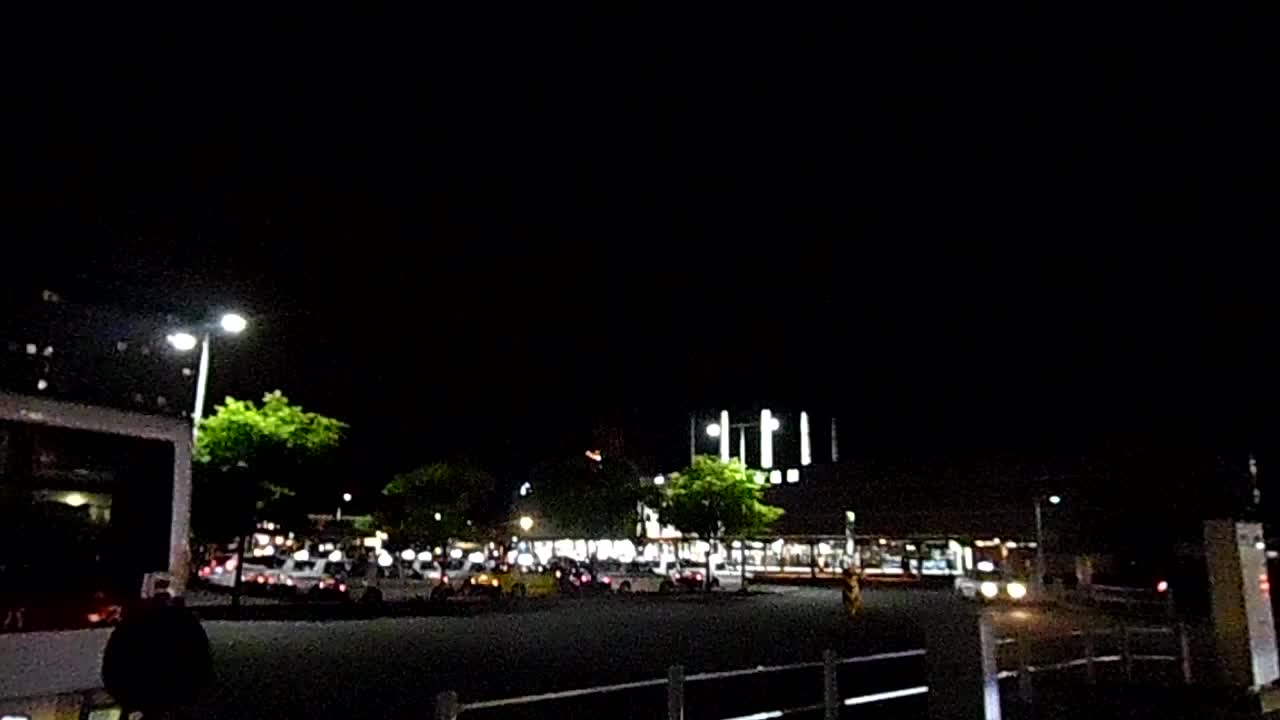This color photograph, captured outdoors at night, showcases a city scene under a pitch-black sky devoid of stars. The image is slightly blurry, making it challenging to discern specific details, but offers a broad perspective of a busy urban area. The primary focus is a large building in the background, emanating a soft white light through its windows, resembling a station or a significant city structure, possibly with some tower-like vertical lights. In front of this building, a well-lit parking lot filled with several rows of parked cars is visible. Among these vehicles, a few yellow cabs are distinguishable, with the rest appearing to be mostly white. Thin, scattered trees punctuate the parking area, along with a fountain and streetlights that provide additional illumination. The image suggests the presence of police patrol cars or a possible convoy heading towards an event, inferred from the brake lights of some vehicles and the general setup. The bottom right corner of the photograph includes a metallic railing, while the left side features a prominent streetlight. Overall, this night scene is framed by sporadic streetlights, stadium-like spotlights, and urban elements, hinting at a bustling yet serene nocturnal cityscape.